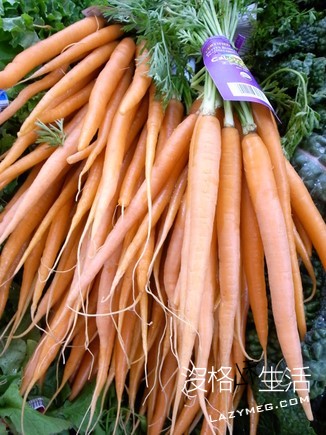The image features an up-close photograph of several bunches of medium-sized, wild-grown carrots with long, thin, string-like roots and vibrant orange color with white-ish shoots. The carrots are bundled together at the top with visible green stalks, which appear fresh and clean, typical of produce seen at a marketplace. Attached to the green tops is a purple label that includes a barcode and some unreadable text. The carrots are laid out on a bed of greens, which might be other vegetables like lettuce, parsley, or cabbage. In the bottom right corner of the image, there are Asian characters and the website name "lazymeg.com" written in small white lettering, suggesting the marketplace might be in Asia.